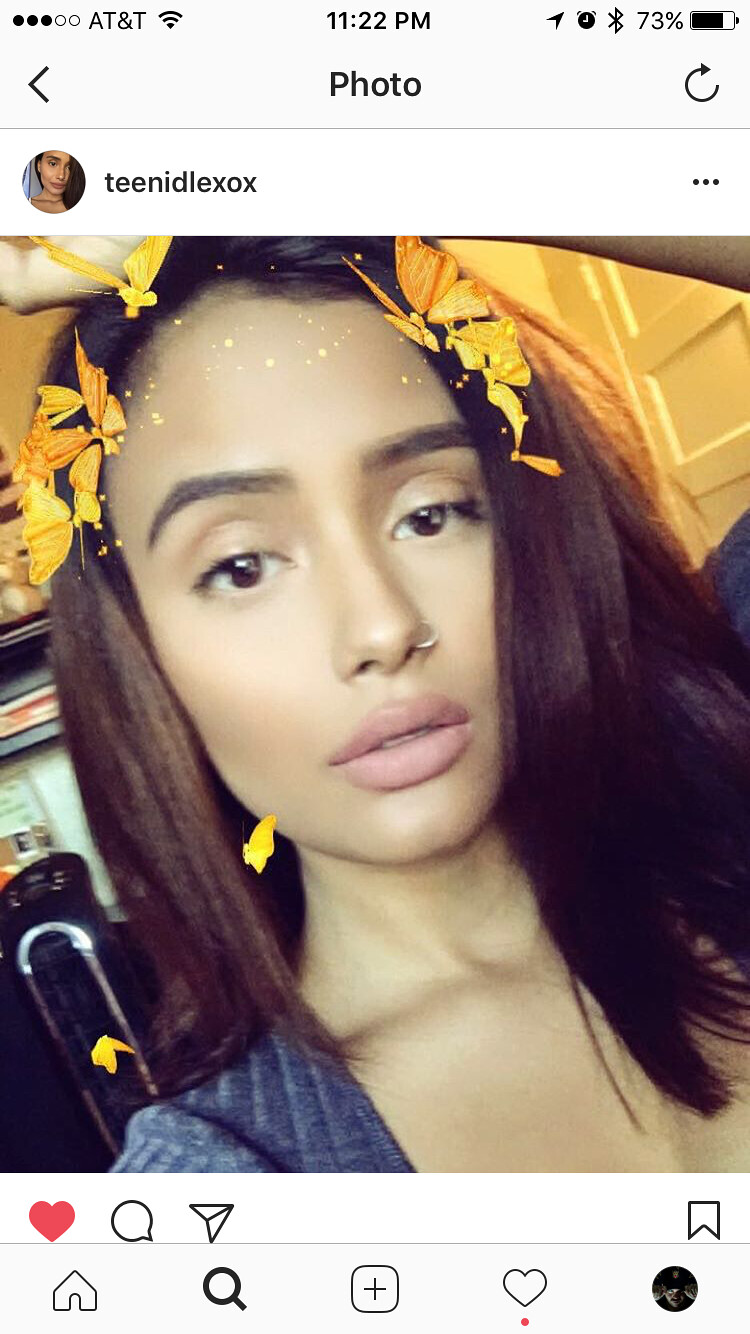This detailed image description portrays a screenshot from a mobile phone displaying a Facebook post by a user named T-E-E-N-I-D-L-E-X-O-X. At the top of the screen, the status bar indicates the carrier is AT&T, the time is 11:22 p.m., and the battery level is 73%. Additional icons on the right include Bluetooth, battery, and signal strength indicators.

The main content beneath this status bar is a Facebook post predominantly featuring a photo of a young woman with dark skin and dark brown hair that falls to her shoulders. She is wearing a blue shirt and has a nose ring. Her lips are plump and slightly parted in a seductive manner. The woman appears to have applied a filter that adds cartoonish, orange butterflies fluttering around her head. The photo seems to be a selfie taken at an angle, slightly tilted. In the background, part of a room is visible, including walls and possibly an exercise machine.

To the left of the woman's name, which is displayed as "teenidlexox," there's a thumbnail image, and to its far right are three vertical dots representing a menu. Below the main photograph, social media interaction icons are visible: a red heart for likes, a comment bubble, a share arrow, and a save bookmark icon. At the bottom of the screenshot, typical mobile navigation icons can be seen, including home, search, post, notifications, and the user profile icon.

Overall, the screenshot portrays a blend of profile information and an aesthetically enhanced, filtered photo presented in a way typical for social media platforms.